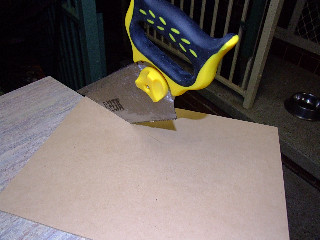In this indoor photo, a yellow-and-blue-handled handsaw is partially embedded in a thin beige sheet of what appears to be plywood. The plywood is positioned on a gray table, possibly made of marble or another hard material, with the board hanging off one side. The silver saw blade, marked with some illegible black writing, is stuck mid-cut within the plywood. The surrounding scene reveals more details: to the right of the image, a silver dish, likely meant for a dog or cat, rests on a carpet that seems to lead either back inside or into another room. In the background, a gray fence or grate is visible, giving the impression that the area might be adjacent to an outdoor deck. Beyond this, another doorway or gate can be seen, though what lies beyond remains obscured by darkness.